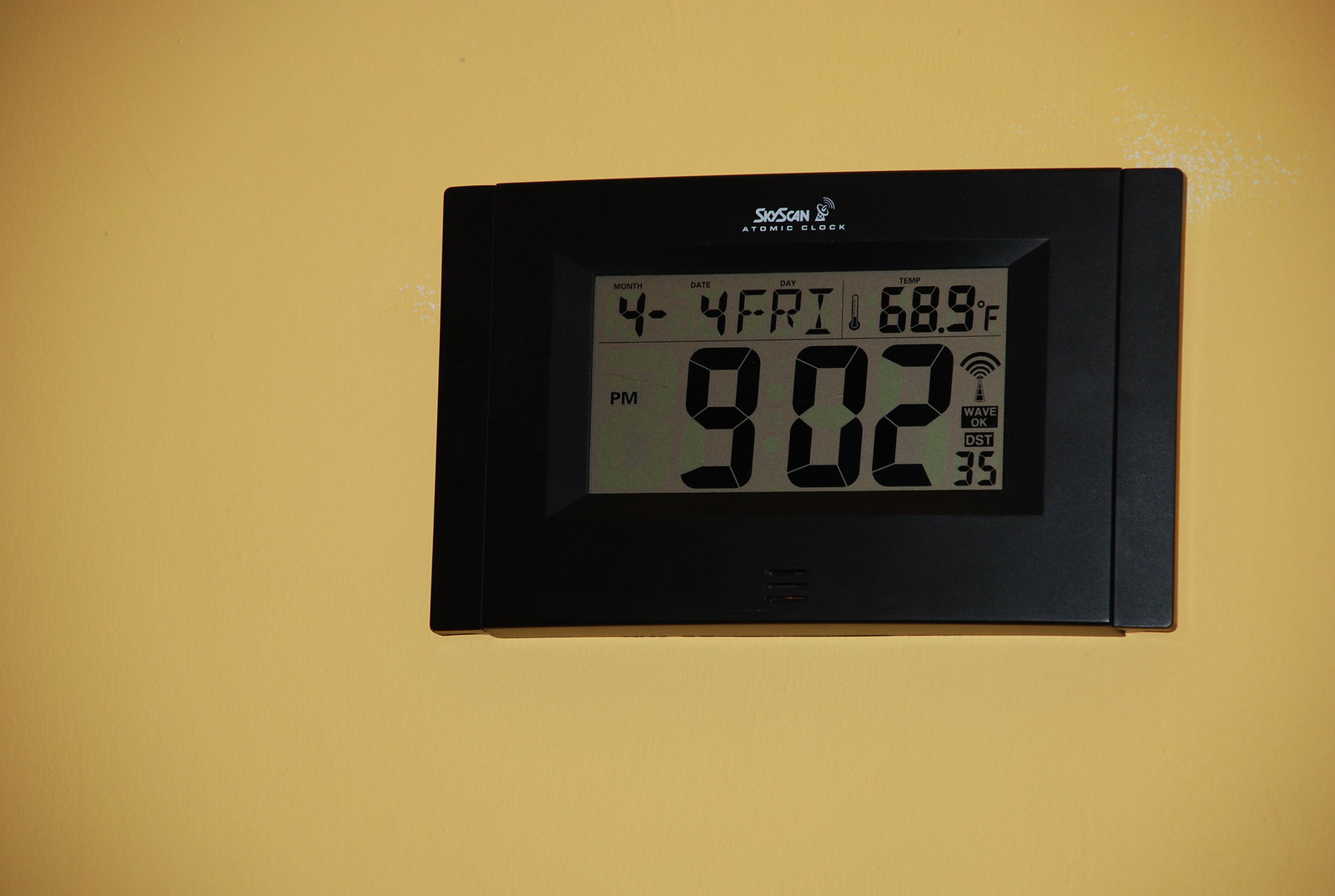The image displays a multifunctional digital device that integrates temperature, time, and date information. The unit is black and rectangular in shape. The brand name, though difficult to discern, appears to be "SoScan" or "SeoScan." Prominently featured on the screen is a radar-like graphic along with the label "Atomic Clock." The readout details the current date as Friday, April 4th, with the temperature at 68.9 degrees Fahrenheit, indicated by a small thermometer icon. The device also shows the current time as 9:02 PM. Additional icons include a Wi-Fi symbol accompanied by the text "Wave OK," and below that, the initials "DST" followed by the number 35. The background of the image is plain, drawing full attention to the device's display.